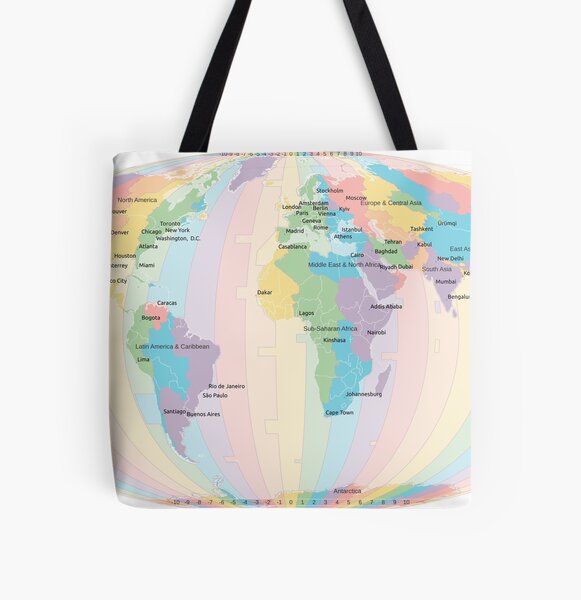The image features a square canvas tote bag set against a white background, adorned with a map of the world. The bag showcases a vibrant rainbow-colored map, with each continent—North America, South America, Europe, Asia, Africa, and Antarctica—depicted in distinct colors such as blue, purple, pink, yellow, and green. The continents are separated by lines of longitude, which include numerical markers ranging from negative 10 to positive 10 meeting at zero in the center. The map displays various cities and countries, each in different colors, creating a striking multicolored effect. The tote bag has sturdy black straps, with the lower portions of the straps visible in the image. There is a white band at the top of the bag where the strap attaches.